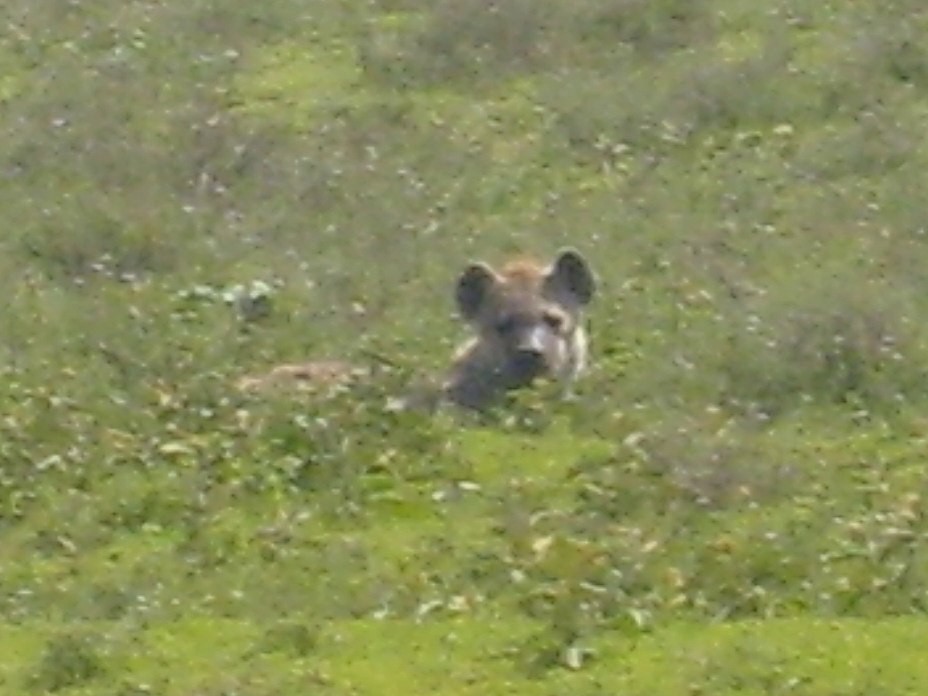In the center of a slightly out-of-focus and grainy image, a brownish wild animal with dog-like ears and a short muzzle, resembling either a honey badger or a hyena, peeks through a dense expanse of green grass in a vast grassland or forest during the daytime. The animal, distinguishable by its brown coloration with hints of blackish gray, stares directly at the camera with a serious expression, while only its head and the top of its body are visible amidst the lush and varied shades of green vegetation surrounding it.